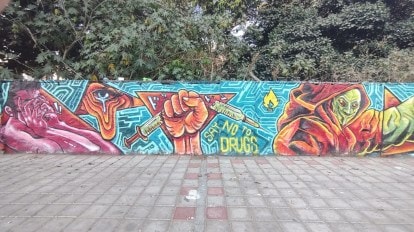The image features an outdoor photo of a graffiti-covered wall set against a backdrop of green trees. The ground in front of the wall is a brick or stone pathway, predominantly light gray with some scattered red squares. The graffiti art spans the entire length of the wall, which has a bright teal blue background with geometric shapes and messages.

Starting from the left, there is a pink-skinned man with dark hair who appears distressed, covering his face with his hands. Next to him is an eye, deeply illustrated with pronounced eyelashes and dripping tears, giving a sense of sorrow or hallucination. In the center of the mural, a clenched fist is vividly depicted breaking a hypodermic needle in half, accompanied by the bold yellow text, "Say no to drugs." On the right side of the wall, a figure resembling an alien or monster is painted with a green face and dressed in a red robe. Adjacent to this figure are additional small white symbols scattered against the blue background, adding more depth and intrigue to the artwork. The entire scene appears to have been taken on a sunny day with some shadows present, highlighting the vivid colors and details of the graffiti.